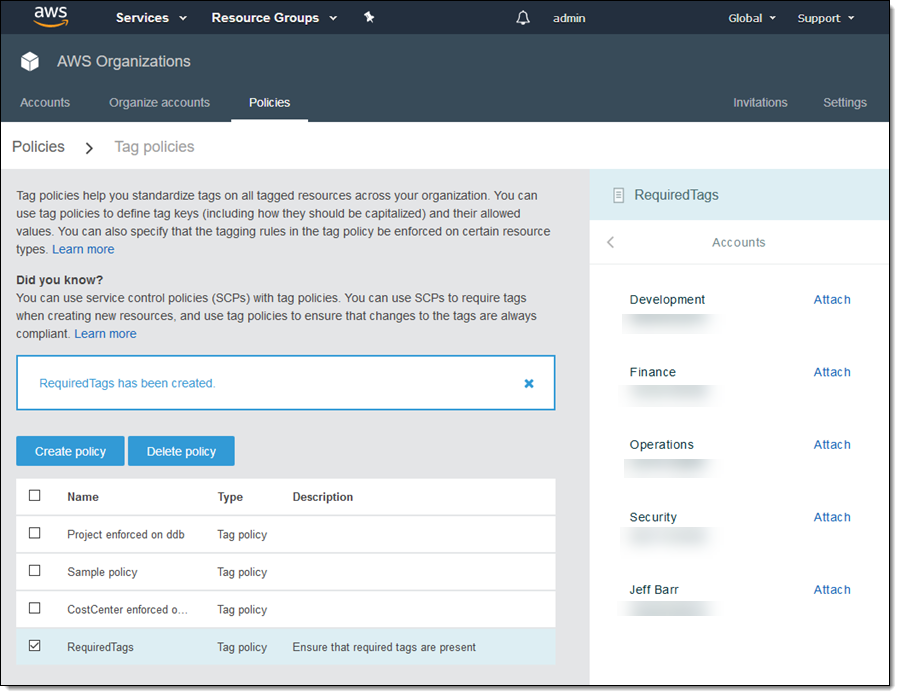Screenshot of AWS Website Interface:
In the top left corner of the screen, the "AWS" logo is displayed in white font with the iconic Amazon arrow underneath, colored in orange. To its right, there are several options, starting with "Services," and "Resource Groups," both in white font accompanied by a white toggle-down arrow. Following these options, there's a shaded white pin icon, a bell icon (not shaded), and "admin" label. Additionally, there are "Global" (unbolded) with a toggle-down option, and "Support" with a toggle-down option next to them.

Below this top navigation, in a slightly lighter blue box, the title "AWS Organizations" appears in white font. Underneath, there is a menu list comprising "Accounts," "Organize Accounts," "Policies," "Invitations," and "Settings," in that order.

Proceeding further down, the screen lightens to a pale gray background with a section titled "Policies" and a sub-option "Tag Policies" beneath it. This area features a grey-shaded section listing various policies with an actionable option for each. Additionally, there are two blue buttons labeled "Create Policy" and "Delete Policy." 

On the right side of this section, under "Required Tags," there are options such as "Development," "Finance," "Operation," "Security," and "Jeff Barr," each with an "Attach" option in blue text next to them.